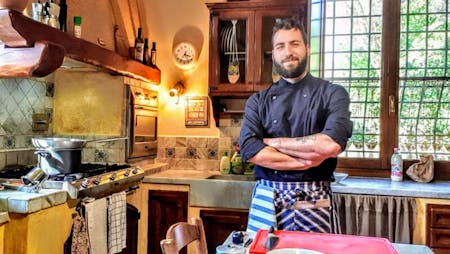The image captures a scene in a well-lit, traditional kitchen, likely in a home, with a man standing confidently at the center. He is smiling warmly at the camera, exuding a sense of pride and hospitality. The man, who has a well-kept brown hair, a full beard, and mustache, is dressed in a black chef’s coat and appears to be tying an apron at his waist, supplemented with multiple towels or a cooking belt, suggesting his professional culinary skills.

His arms are crossed in front of him as he poses in front of a sturdy wooden table with a pink cutting board and a knife placed atop. In the foreground is a wooden chair. To the left of the man is the kitchen’s stove, which holds a pot and a skillet, adding to the lived-in and actively-used feel of the space. Above the stove is a shelf stocked with various spices and glass bottles, providing a glimpse into the culinary tools and ingredients at the man’s disposal. 

The kitchen is adorned with practical and homey elements: a wall hanging beside a light bulb that illuminates the room, a nearby white clock, and a shelf housing assorted kitchen utensils. Behind the man, large brown-framed windows reveal a view of lush trees, indicating the kitchen's integration with its natural surroundings. The room features partial tiled walls and marble countertops, adding to its traditional yet functional charm. Additional details such as a microwave near the windows and liquid soap on the kitchen counter highlight the blend of professional and home kitchen elements, enhancing the scene's authenticity.